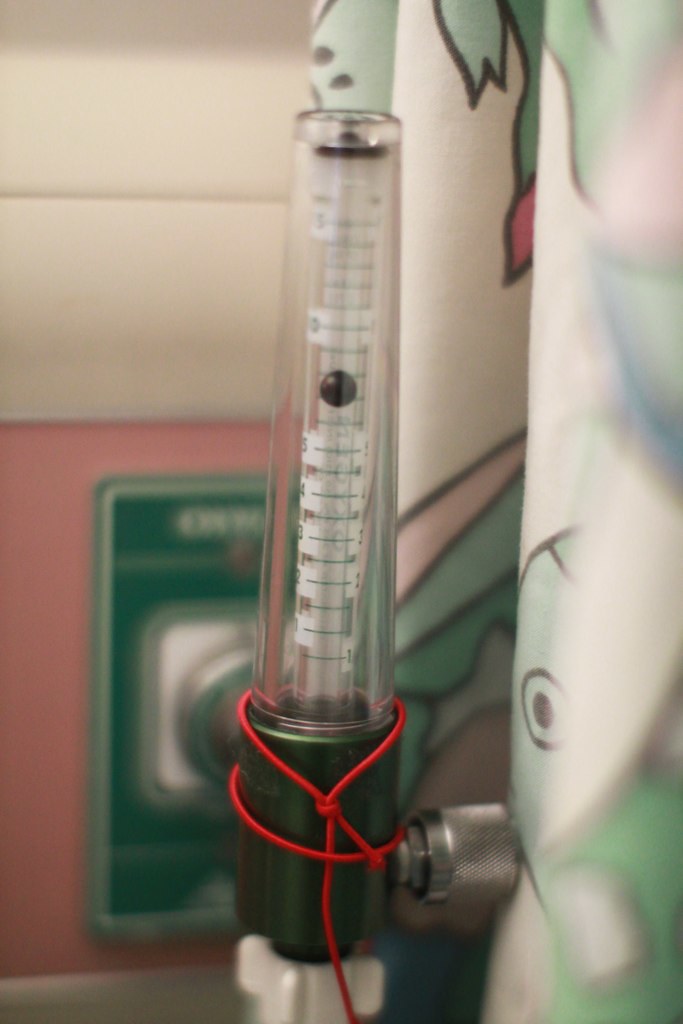The image depicts a vertical measuring device that closely resembles a thermometer, mounted within a clear plastic tube. The bottom portion of the apparatus is green and is secured by a very thin red cord. Inside the transparent casing is a slender measuring stick featuring a white background with black notches, although the exact numbers are not discernible. A small black dot is suspended midway along the length of this vertical apparatus. To the left of the device hangs a curtain adorned with white, green, and light pink patterns. Adjacent to the curtain, there is a green and white knob or sign affixed to a wall that is painted in shades of pink and white. The entire setup suggests that the device might be used for measuring some form of flow, although the exact nature of what is being measured remains unclear. The setting, along with the specific design cues, hints that this could be located in a hospital environment.